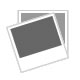In a landscape-oriented image with a bright blue background, a person’s hand emerges from the bottom-left corner, holding an electronic measuring device resembling a micrometer. The device, primarily black, features a digital reader displaying "50.28 millimeters." It includes several buttons: a red "On/Off" button, a yellow "Zero" button, and a blue button labeled “mm/inch/F.” Alongside the measuring instrument, metallic slats and a dark metal part with screw holes are visible, suggesting the measurement of an automotive or engine component. At the top of the image, a black banner reads "W.O.R.P. White Oak Race Products" accompanied by five gold stars and the text "Fast Shipping - Easy Returns."